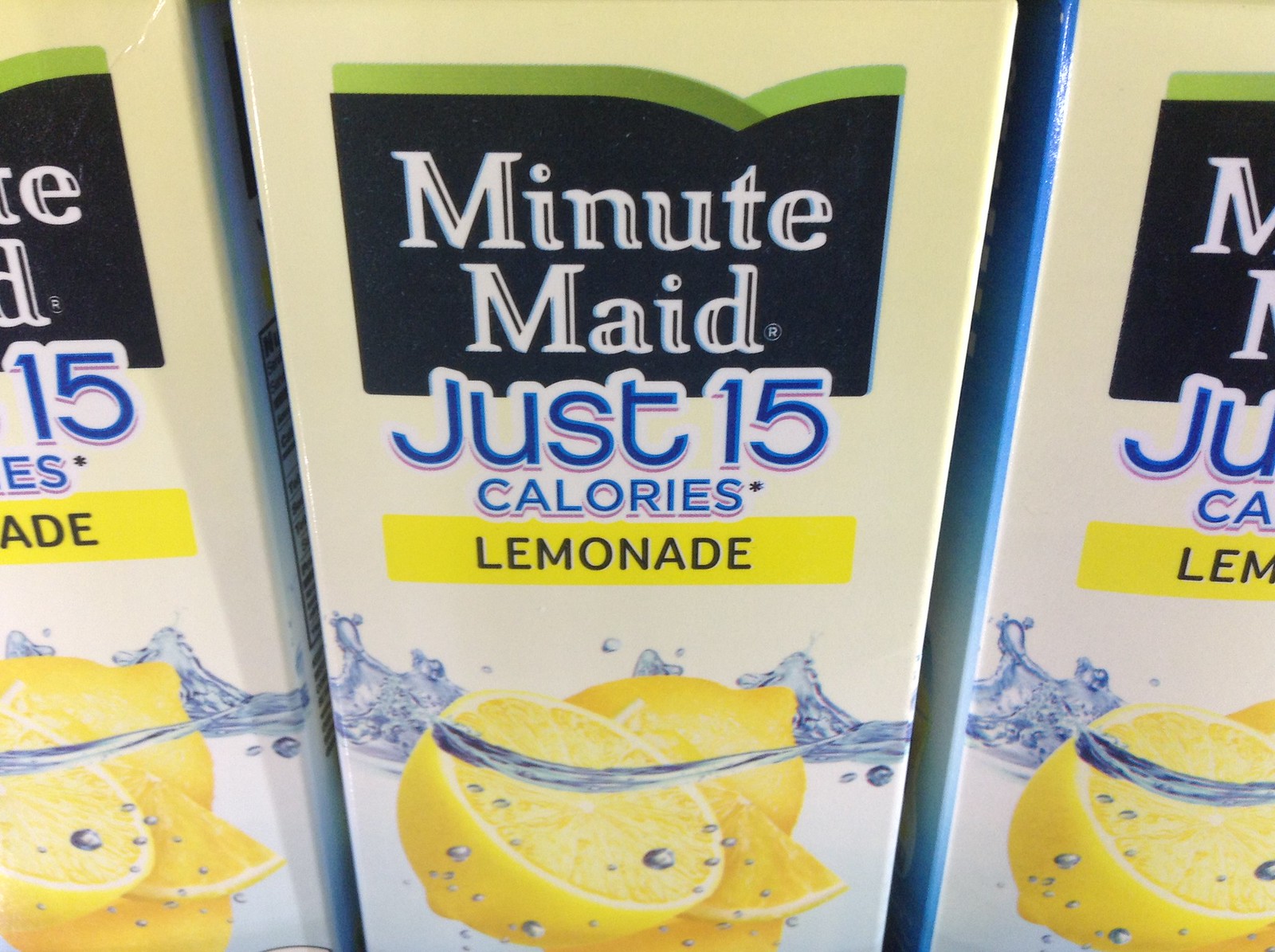This image is a close-up shot of three Minute Maid lemonade bottles positioned on a shelf in the cold section of a store. The bottles are styled similarly to old-school milk cartons with a beige color. The prominent Minute Maid emblem is displayed at the top, featuring a black background with a green border. The "Minute Maid" text is white with highlighting, giving it a 3D effect. Below this, there is text in blue stating "Just 15 Calories," and a yellow square containing the word "Lemonade" in black. The packaging also includes images of sliced lemons in water. The perspective of the photo partially cuts off the top and bottom of the bottles. The first and third bottles are only visible halfway down, indicating they are arrayed closely on the shelf.